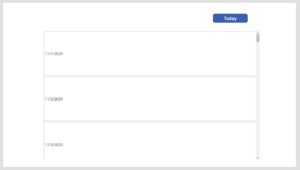The image depicts a screenshot set against a clean white background. Dominating the view is a prominent blue rectangle with the word "Today" displayed in white text. Below this are three smaller rectangles, each containing a single word that is unfortunately too small to be legible. To the right side of the image, near the top corner, there is a visible gray scroll bar, indicating that additional content can be accessed by scrolling. The overall layout suggests an interface, possibly from a digital application or a web page designed for efficient navigation and readability.